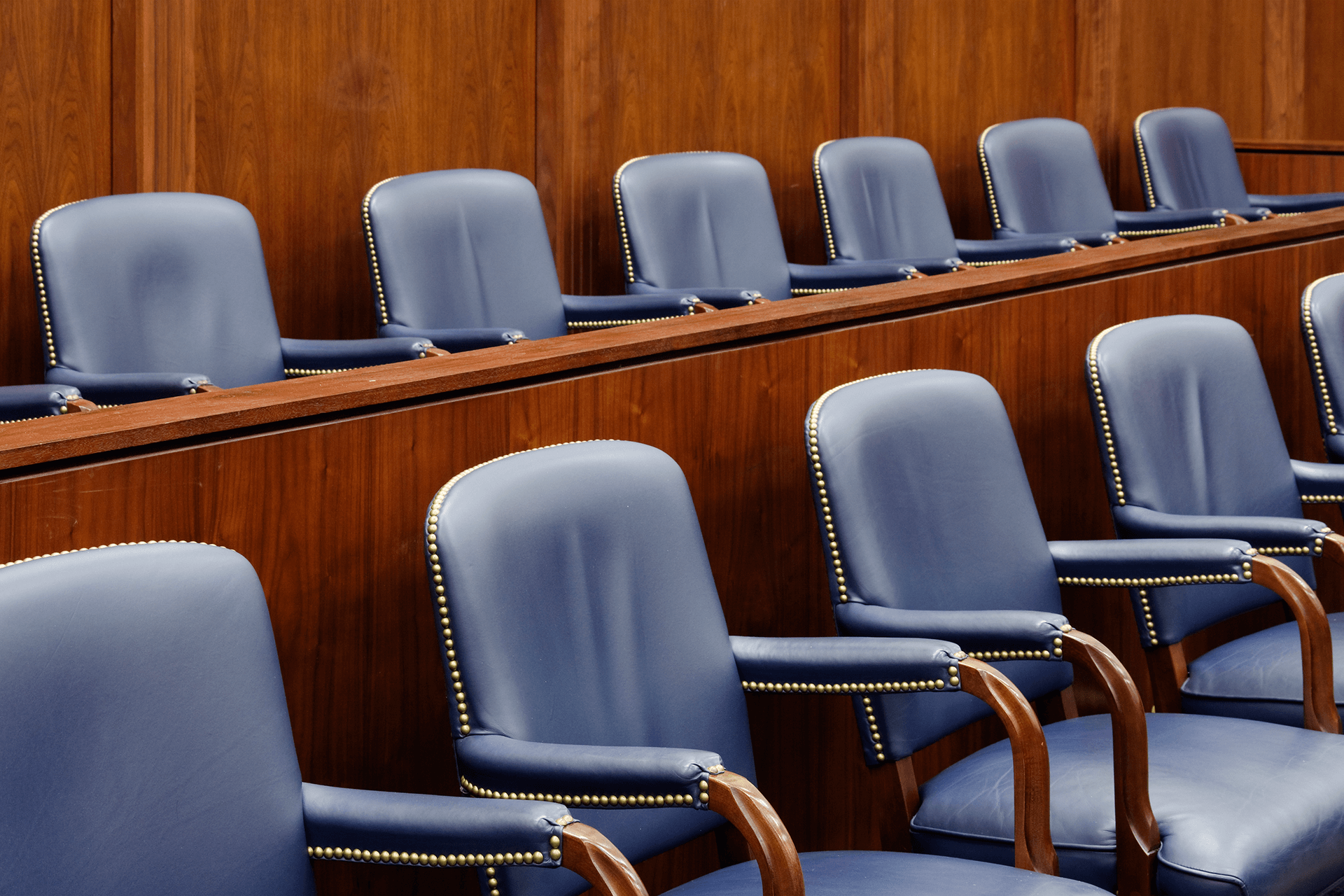The image depicts a section of what appears to be a courtroom, possibly a jury box. The scene shows two rows of leather chairs, arranged in a setting typical of official or government buildings. In the back row, there are seven seats, with one partially obscured on the far left, and the front row comprises five seats. The chairs are upholstered in a dark blue, almost black, leather, featuring a pattern secured by circular gold studs. The hand rests of the chairs are also wrapped in the same leather. The backdrop is a wall with a medium-tone brown wood stain, adding to the formal ambiance of the space. The raised area behind suggests an elevated positioning, characteristic of a juror's seating arrangement. The area is devoid of people, emphasizing the orderly alignment of the chairs.